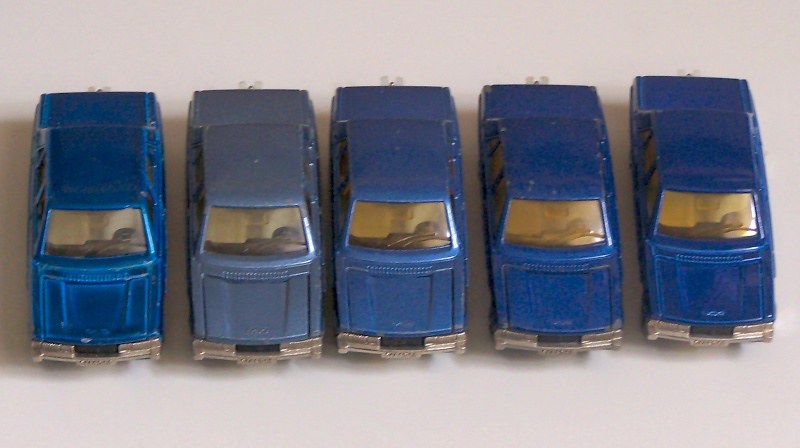This photograph captures a top-down view, angled slightly forward, of five blue toy sedans arranged in a neat row on a white surface. The toy cars appear to be identical in model, each with a squared and angular body design, featuring chrome bumpers and placeholder spots for headlights. Despite their identical shapes, the cars display variations in their shades of blue due to wear and age. The first car on the left stands out with a vivid blue color, followed by a faded pale blue car, then a slightly deeper blue in the middle, and concluding with two more blue cars that, while not as vibrant as the first, are nonetheless more vivid than the paler one. The windshields on these cars are reflective, with hints of a yellowish tint, resembling a mirror finish. This assortment of toy cars, reminiscent of Matchbox cars, showcases slight color inconsistencies, adding a nostalgic charm to their orderly presentation.